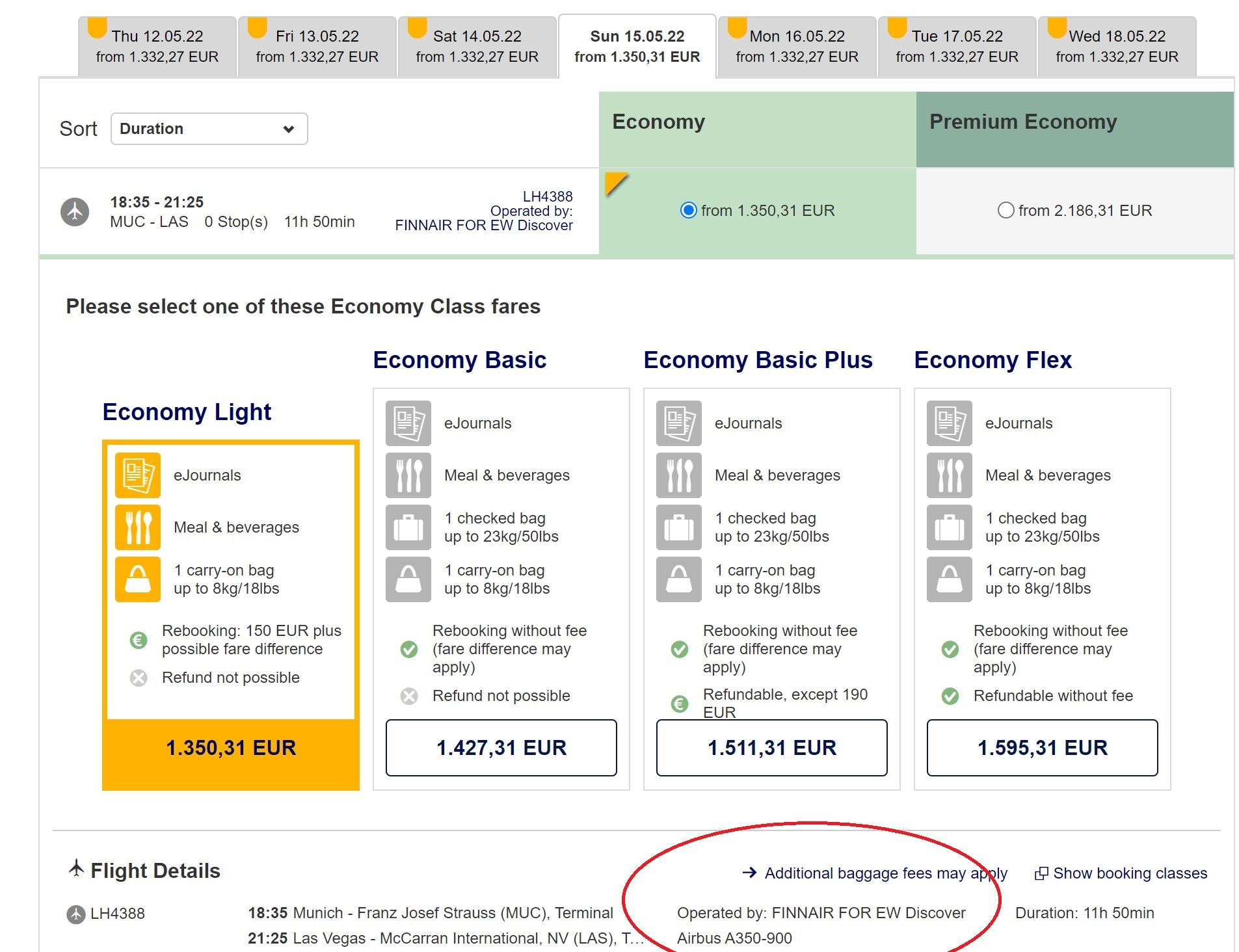**Flight Details: MUC to LAS**

- **Flight Duration:** 11 hours, 50 minutes
- **Flight Number:** Operated by Finnair for EW Discover
- **Flight Route:** Munich (MUC) to Las Vegas (LAS)
- **Aircraft:** Airbus A350-900

**Class Options and Pricing:**

- **Economy:**
  - **Basic:** Starting from 1,350.31 EUR
    - Includes: 
      - E-Journal access
      - Meals and beverages
      - One checked bag up to 23 kg (50 lbs)
      - One carry-on bag up to 8 kg (18 lbs)
      - Rebooking without a fee (fare difference may apply)
      - Non-refundable
  - **Basic Plus:** 1,427.37 EUR
    - Note: Additional baggage fees may apply

- **Premium Economy:**
  - Starting from 2,186.31 EUR

**Class Options and Pricing (Economy Class):**

- **Basic:**
  - Includes:
    - E-Journal access
    - Meal and beverage service
    - One checked bag up to 23 kg (50 lbs)
    - One carry-on bag up to 8 kg (18 lbs)
    - Rebooking without a fee (fare difference may apply)
    - Refund not possible
  - Price: 1,427.37 EUR

**Additional Notes:**

- All provided information, including pricing, is clearly highlighted and marked for emphasis with a red circle in the original document.